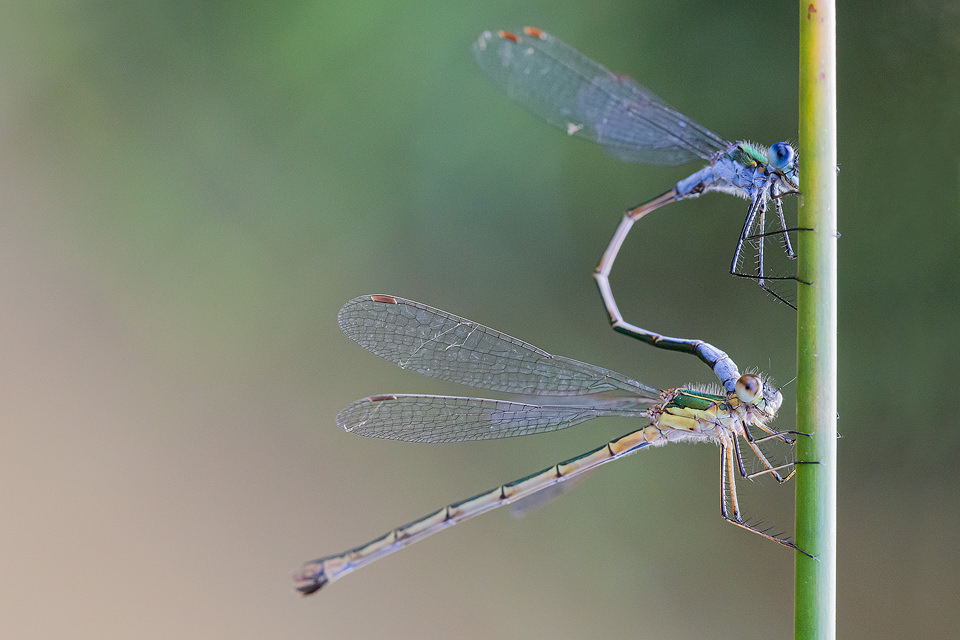This close-up daytime photograph captures an intimate moment between two dragonflies perched on a vertical green twig, likely situated in a garden. The background is artistically blurred, showcasing a palette of greens and hints of pinks that suggests a serene, natural setting. Against this softened backdrop, the dragonflies stand out with their bluish-gray wings and elongated bodies. One dragonfly sits above the other, its tail gracefully curled into an S-shape and touching the back of the lower dragonfly's head, possibly hinting at a mating behavior or form of communication. The detailed structure of the twig and the precise positioning of the dragonflies create a visually striking and intriguing scene.